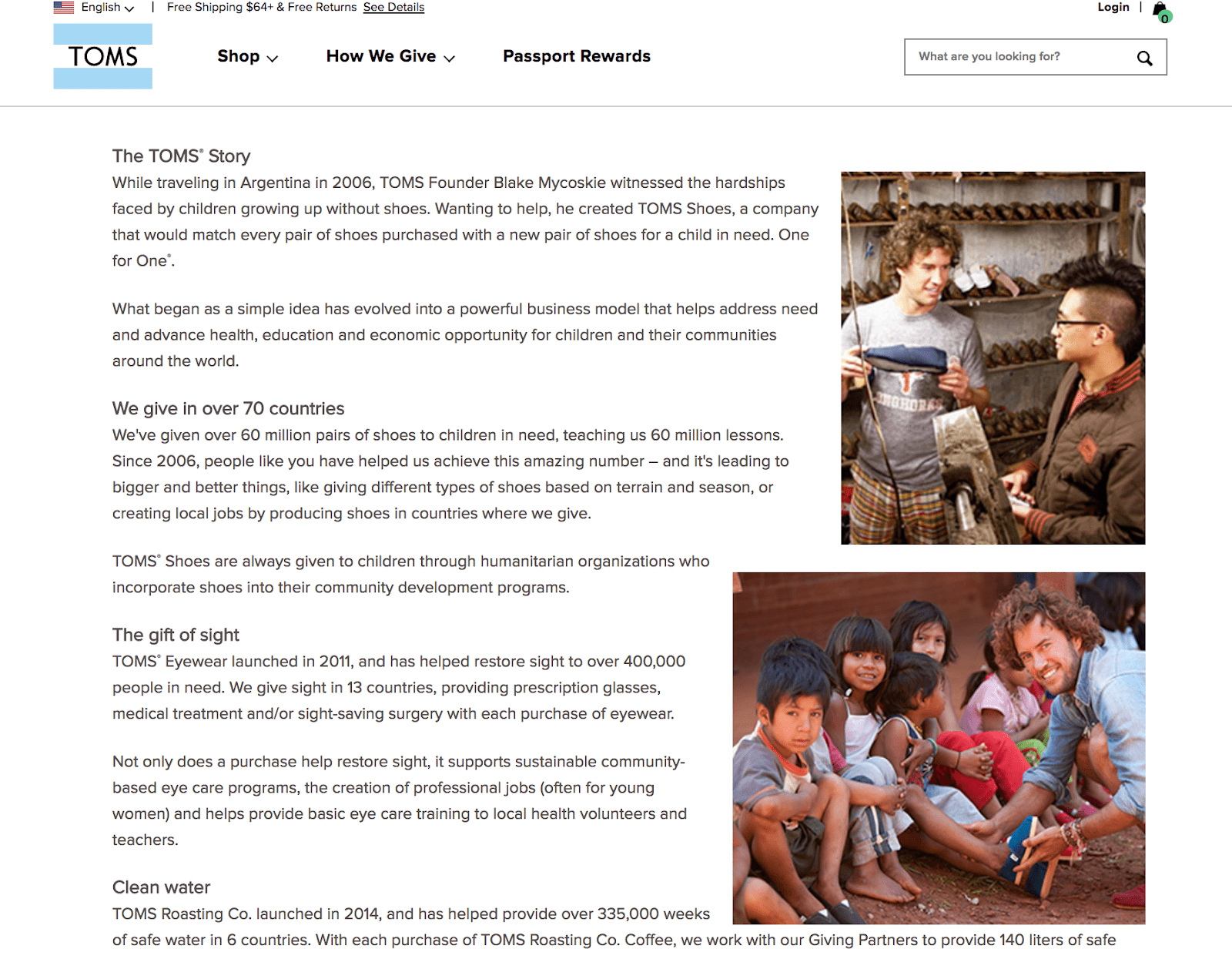In this article from TOMS' official website, the clean and user-friendly layout includes a search bar on the right and an option to select different languages. The story of TOMS, prominently featured, recounts how the founder, Blake Mycoskie, was inspired to create the company during his travels in Argentina in 2006. Moved by the difficulties faced by children growing up without shoes, Mycoskie established TOMS Shoes with a unique business model: for every pair of shoes purchased, a new pair would be given to a child in need, following the "One for One" philosophy. 

The company's charitable efforts have extended to over 70 countries. In 2011, TOMS Eyewear was launched, dedicated to restoring eyesight for those in need, impacting over 400,000 individuals to date. Further details include programs aimed at providing clean water. On the right side of the webpage, two pictures of Blake Mycoskie are displayed. The top image captures him showcasing a pair of TOMS shoes to a young Asian man with a mohawk and glasses in a shoe store. In the bottom image, Mycoskie is seen in a modest village in Southeast Asia, surrounded by joyous children sitting on the ground. Mycoskie appears to be a Caucasian man in his 30s, visibly engaged in the community's daily life.